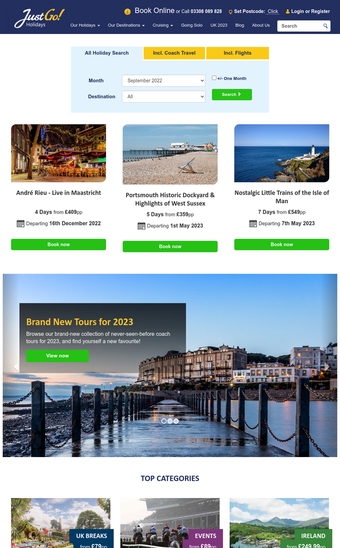The advertisement showcases a travel-style website with a sleek and inviting design. At the top, a navy-colored banner prominently displays the slogan "Just Go." It includes key navigation features such as options to "Book Online," set a postcode, and buttons for "Login" or "Register." Below this, easy-to-access links to "Our Holidays" and "Our Destinations" are listed, alongside a well-positioned search bar. Additional navigation includes clickable links for "Blog" and "About Us" pages. 

The search bar is customized with options to search for holidays by month—specifically "September 2020"—and destination, with a standout green "Search" button. Visitors can refine their search to include coach travel or flights. Below the search functionality, the advertisement features three enticing images: the first depicts a serene beach with a distant pier; the second showcases a scenic mountainside overlooking the ocean; and the third captures a vibrant city festival scene, highlighting "Andre Rieu live in Maastricht."

Additional features include specific destination highlights like the "Portsmouth Historic Dockyard," "Highlights of West Sussex," and the "Nostalgic Little Trains of the Isle of Man." The ad promotes "Brand New Tours for 2023," urging users to explore a fresh collection of never-before-seen coach tours. The website also invites users to discover new favorite views with categories like "Top Categories: UK Breaks," "Events," and "Ireland" listed as travel options.